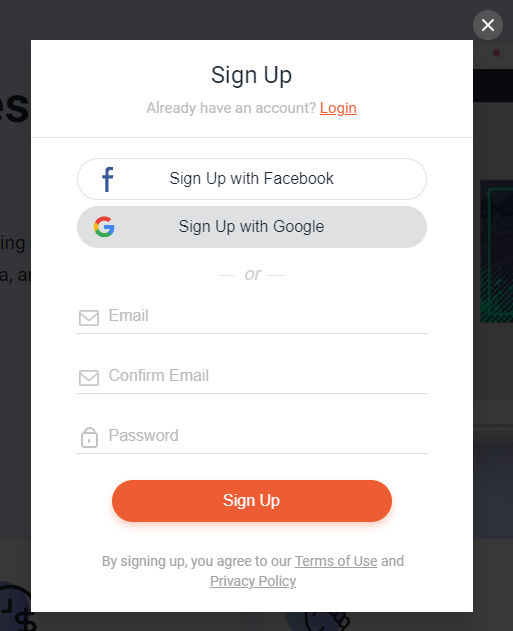This image captures a signup window for a website, prominently featuring a blue rectangular box with various elements. At the top right corner of the image, there's a white 'X' enclosed in a gray circle, likely a close button. The background contains a partially obscured website, making it difficult to determine its content.

The main section is dominated by the blue box, which has the title "Sign Up" in black at the top. Just beneath this, in light gray text, it reads "Already have an account?" followed by an orange "Login" option.

A horizontal line divides the next section, which features two oval-shaped buttons stacked vertically. To the left of the top button, there's the Facebook icon, accompanied by the text "Sign up with Facebook." Below that, the Google icon is displayed next to the text "Sign up with Google."

Further down, there are three input fields labeled "Email," "Confirm Email," and "Password." The "Email" and "Confirm Email" fields both have an email icon next to them, while the "Password" field has a lock icon.

At the bottom of the blue box, there is a green oval button with the word "Sign Up" in the center. Underneath this button, it states in smaller text, "By signing up you agree to our Terms of Use and Privacy Policy."

Overall, the image clearly illustrates the various steps and options available for user registration on the website.